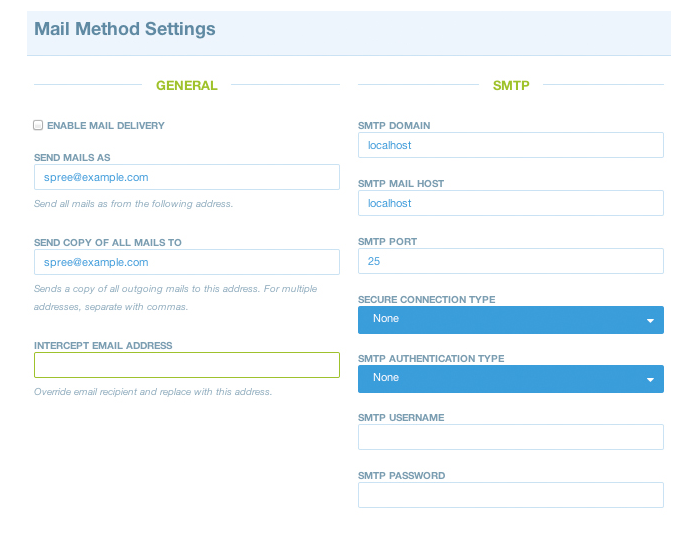Here is a detailed and cleaned-up caption for the image described:

---

This image is a screenshot of an email settings page, likely from a website due to its categorization. The interface features a light blue banner at the top with the text "Mail Method Settings" in a darker blue font. A column on the left is labeled "General" in green font, offering various configuration options:

- A checkbox labeled "Enable mail delivery" is present.
- Below this is a fill-in box labeled "Send mails as," currently set to "spree@example.com." The description clarifies that this address will be used for sending all emails.
- Another fill-in box, labeled "Send copy of all mails to," is also set to "spree@example.com." The accompanying description explains that a copy of all outgoing emails will be sent to this address and multiple addresses can be separated by commas.
- There is a highlighted fill-in button next to "Intercept email address," indicating it will override the email recipient and replace it with the specified address.

On the right, there is an "SMTP" column featuring several settings:
- "SMTP domain" and "SMTP mail host" are both set to "localhost."
- "SMTP port" is configured to "25."
- There is a drop-down menu for "Secure connection type," with "None" selected.
- Another drop-down menu for "SMTP authentication type" also has "None" selected.
- Both "SMTP username" and "SMTP password" fields are currently blank.